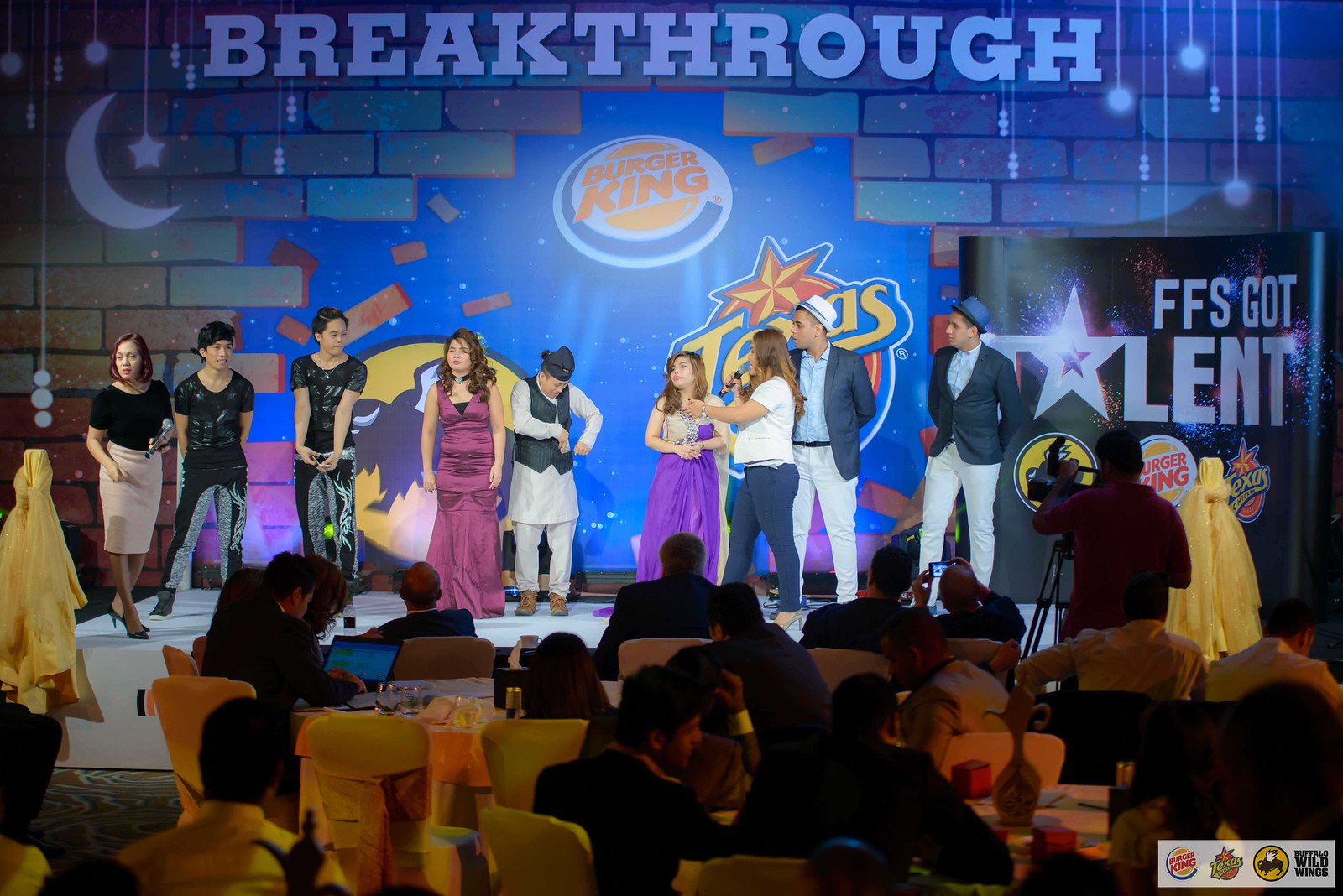The image depicts a vibrant talent competition scene, likely themed as "FFF's Got Talent," with nine participants on stage, all dressed in a variety of costumes ranging from princess dresses to casual shirts and hats. A large banner at the top states "Breakthrough," alongside prominent logos of Burger King, Buffalo Wild Wings, and an obscured Texan-themed logo featuring a star. These elements shine through a backdrop designed to look like bricks being broken, revealing a blue sky and a crescent moon. The audience sits at round tables and yellowish chairs, some positioned around a judges' table. To the right, a cameraman films the event, capturing the dynamic atmosphere of this dinner theater setting.